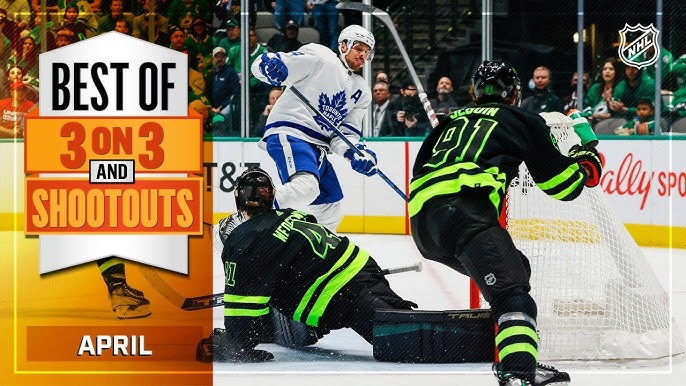In the horizontally oriented image of an NHL hockey game, we see a tense moment of action. The central focus is a goalie, kneeling on the ice, clad in a black jersey with neon green accents and black pants, vigorously defending the goal. Flanking him are two other players: one, also in a black and neon green uniform, is skating nearby, while the other is an opponent from the Toronto Maple Leafs. This player in white and blue, with a blue maple leaf logo and a letter 'A' on his jersey, is poised with his stick, likely attempting to score. The backdrop includes an eager audience behind the glass, intently watching the unfolding action. On the left side of the image, text reads "Best of Three on Three and Shootouts" with "April" just below it, placed over a semi-transparent orange-striped section. The NHL logo is visible in the upper right corner, completing this vivid snapshot of a competitive moment on the ice.